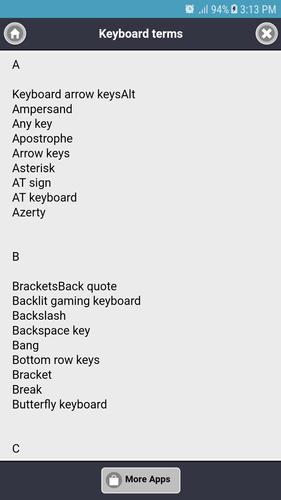The image primarily consists of a screen interface with several distinct sections and details. It is divided into various blocks with a mix of rectangular and circular elements, adorned with text and icons.

At the top of the screen, there is a blue rectangle displaying a clock symbol on the left, with subsequent lines increasing in height from left to right, leading up to a "94%" label next to a battery icon. Further to the right, it indicates the current time "3.13 PM."

Beneath this, there is a more prominent dark blue rectangle. In the center of this dark blue rectangle, there is a light gray circle with a darker gray inner circle that contains an icon of a white house. Adjacent to this, the text reads "keyboard terms." To the right of this circle, there is another light gray circle with a slightly darker gray inner circle that has an X symbol inside.

Continuing below, there is a list beginning with the letter "A," followed by several keyboard-related terms such as "keyboard arrow keys," "ALT," "ampersand," "any key," "apostrophe," "arrow key," "asterisk," "AT sign," "AT keyboard," and "AZERTY."

Next, under the letter "B," the list includes terms like "brackets," "back quote," "backlit gaming keyboard," "backslash," "backspace key," "bang," "bottom row keys," "bracket," "break," and "butterfly keyboard."

Lastly, under the letter "C," the screen shows another dark blue rectangle containing a light gray rectangle. Within this light gray rectangle, there is a dark gray circle featuring an icon that resembles either a house or a shopping bag. The associated text reads "more apps."